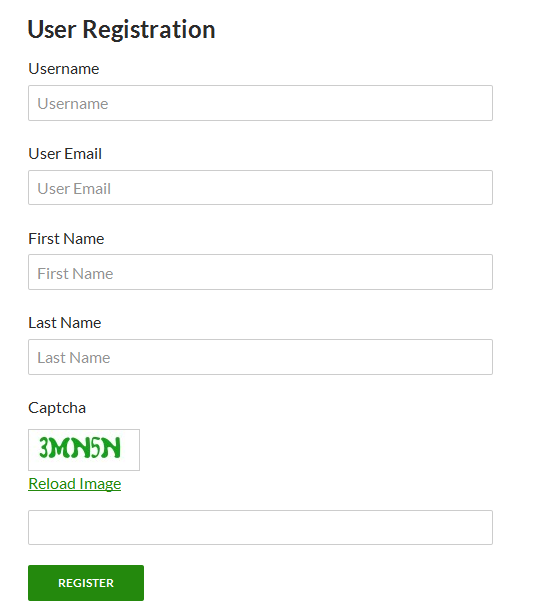The image showcases a user registration page set against a white background. At the top, "User Registration" is prominently displayed in large black font. Below this heading, the form is laid out in a series of labeled fields. The first field is for "Username," with an empty text box to input the user's desired username. The next field is labeled "User Email," also paired with an empty text box for typing in the user's email address.

Following this, there are fields for "First Name" and "Last Name," each with a corresponding text box for entering the respective personal information. Below these, a CAPTCHA section is presented. The CAPTCHA text "3MN5N" is displayed in green, wavy font within a designated box. Adjacent to this is a green "Reload Image" button, allowing the user to generate a new CAPTCHA if needed. Directly beneath the CAPTCHA text, there is an empty text box where users are expected to type the shown characters for verification purposes.

At the bottom of the form, there is a prominent green button labeled "Register" in white font, which users can click to submit their registration details.